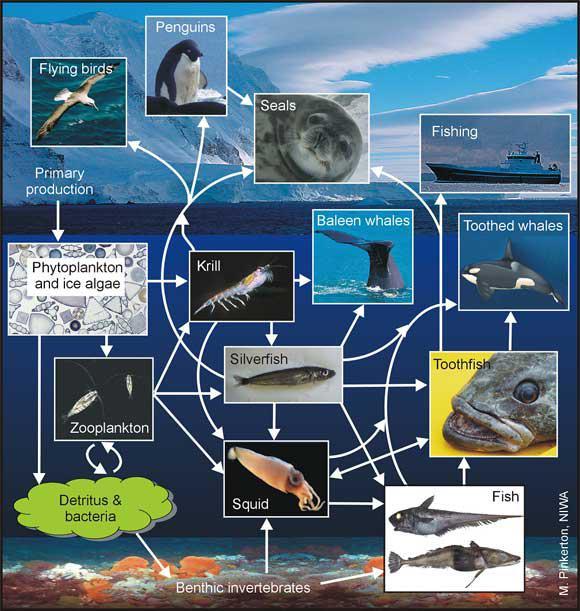This is a detailed infographic poster illustrating the ecological connections and food chains in the Arctic environment, both above and below the water. The background shows a serene ocean scene with a snow-covered mountain and glaciers, setting the context for the Arctic ecosystem. The diagram is structured like a flow chart, with various panels and images superimposed over this scenic backdrop.

At the very bottom of the underwater section, the infographic begins with benthic invertebrates. Above them, primary production is highlighted, featuring phytoplankton and ice algae, which are crucial for sustaining the marine food web. The arrows from these primary producers point towards zooplankton and detritus, indicating their role in the ecosystem. Further up are images of krill, squid, silverfish, and toothfish, each connected by arrows to show the flow of energy and matter.

Above the waterline, the infographic shows a variety of life forms, including flying birds, penguins, and seals, each depicted in individual panels. These panels are interconnected with arrows leading back to their respective prey, such as silverfish, illustrating their dietary relationships. Additionally, a fishing boat is included, symbolizing human involvement in the Arctic ecosystem.

The poster is signed "M. Pinkleton NIWA" and effectively conveys the intricate relationships between different species, from microscopic phytoplankton to majestic whales, through a network of arrows and images that depict who feeds on whom in this cold, yet vibrant, ecological system.